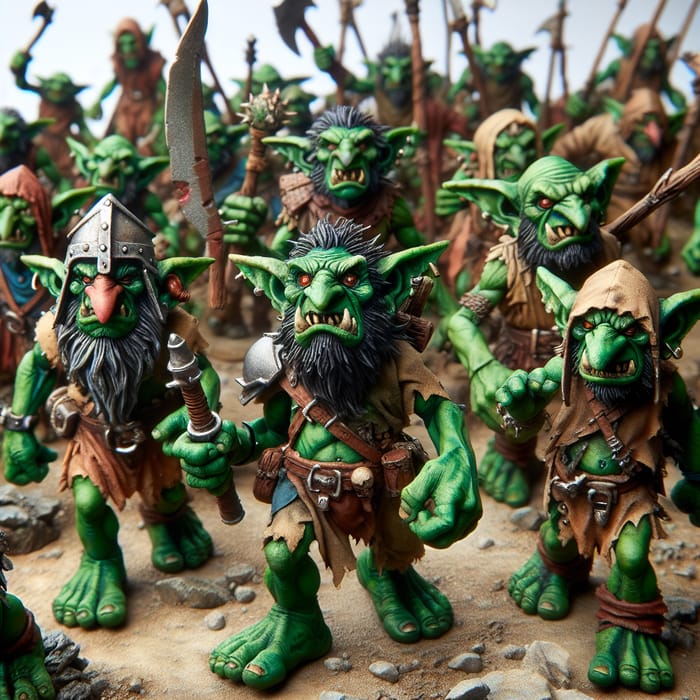This image captures a highly detailed and vivid scene of approximately 20 green Troll figurines, rendered in a 3D style that makes them appear almost lifelike. The Trolls are distinctive with their large, bare feet and massive, oversized hands. Their skin is entirely green except for their fang-like teeth, which jut menacingly from their bottom lips, and their glowing red eyes that add an eerie glow. Each Troll sports snaky black hair and beards, contributing to their fierce appearance.

They are depicted as a marching horde, advancing down a rocky hill, clad in raggedy leather battle clothing and a variety of headgear including helmets, hoods, and some with bare heads featuring long black hair or being bald. They wield an assortment of medieval weaponry such as maces, pikes, halberds, swords, and axes, suggesting they are ready for battle.

Their pointy ears, large pointed noses, and underbites with prominent fangs give them a fearsome look. Despite the minimal clothing, primarily consisting of loincloths, shoulder armor, and leather belts, their muscled green bodies are well-detailed, emphasizing their brutish strength. The scene is set against a rocky, dirt-strewn ground, creating a dramatic and dynamic composition as the Trolls march forward, their expressions filled with rage and determination.